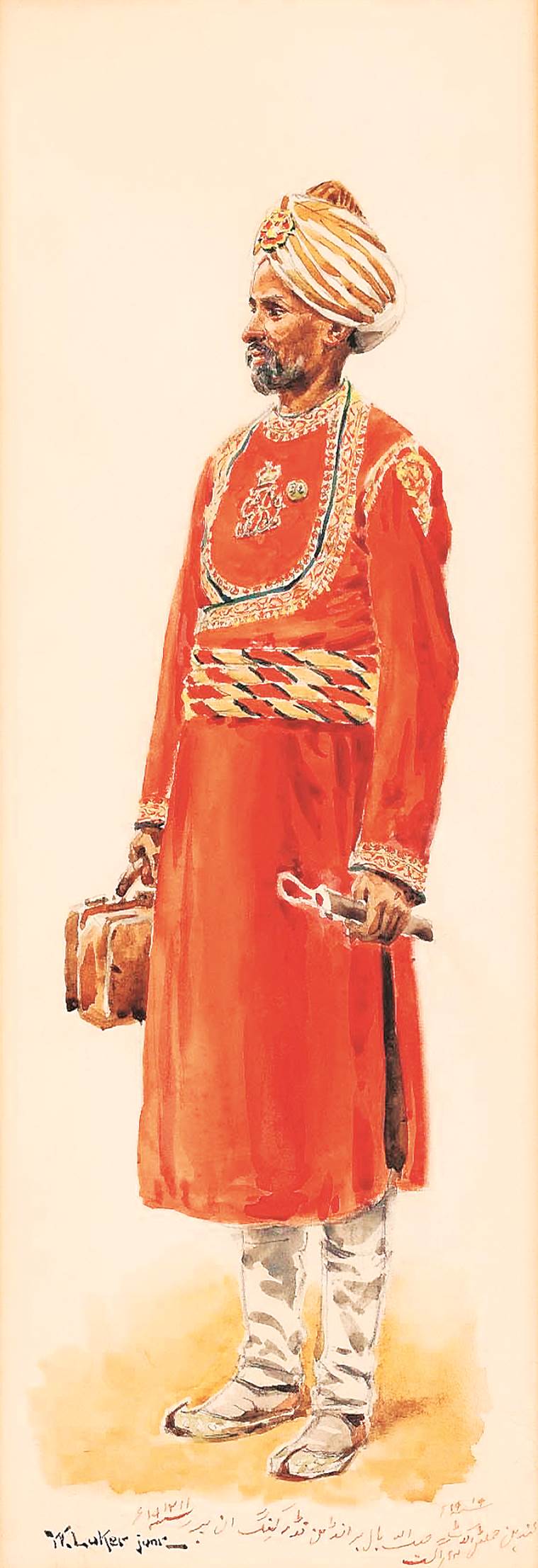This image is a detailed drawing or painting of a man, who appears to be from either a Middle Eastern or Asian background, wearing traditional attire reminiscent of Aladdin’s. The man is standing with his back slightly turned to the right side and his front slightly turned to the left. He is depicted in front of a predominantly pink backdrop, with a subtle shading of brownish-yellow underneath his feet, which suggests ground or dirt.

The man has dark skin and a goatee, along with a white turban adorned with a brooch in the center. His beard shows traces of gray. He is dressed in a knee-length, long red gown with long sleeves. The gown is intricately designed with gold or yellow trim across the chest and around the cuffs, as well as additional embroidery on the bodice and cap of the sleeves. Around his waist, he wears a broad cummerbund featuring a red and golden-yellow pattern, which may include up to four belts of similar coloration.

In his left hand, the man holds a piece of metal, possibly a medical tool like a stethoscope, leading to the speculation that he might be a doctor. In his right hand, he carries a brown bag, perhaps a briefcase or medical case. He also wears white pants and brown shoes, with his right foot slightly turned to the left and his left foot facing straight ahead.